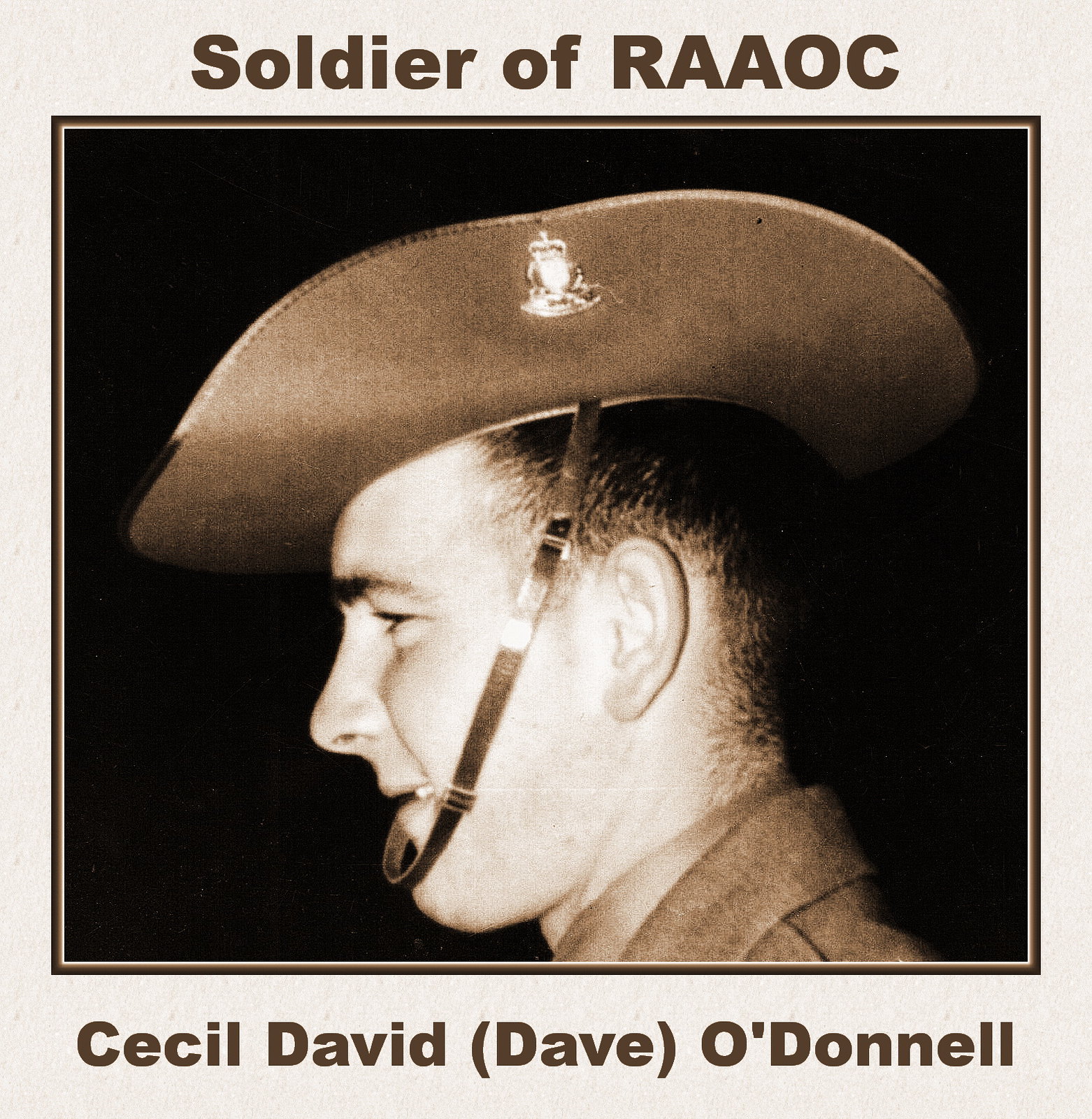This black and white photograph depicts a side profile of a man identified as "Cecil David (Dave) O'Donnell," a soldier of the R.A.A.O.C. The image highlights his distinct military hat, featuring its brim folded up with a strap extending from the top around his chin area, worn loosely near his mouth. The hat also has an emblem located centrally on its left side. The man sports dark, shaved hair and thick eyebrows, without any facial hair, and he is dressed in a uniform. The photograph is enclosed in a light gray frame, with the title "Soldier of R.A.A.O.C." in brown print at the top, and his name, "Cecil David (Dave) O'Donnell," similarly printed at the bottom.